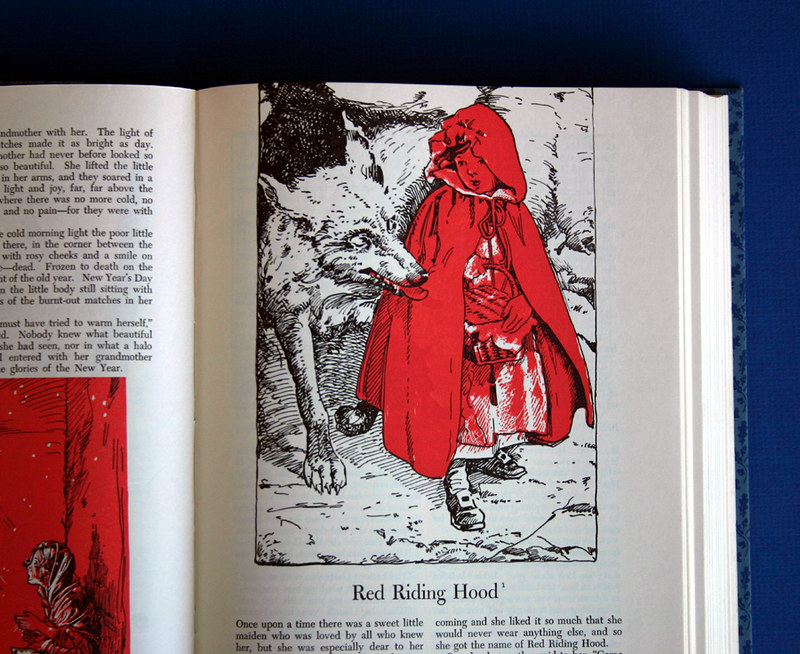The photograph captures an open storybook featuring the tale of Little Red Riding Hood. The left page is partially cut off, displaying black text on a white background in the top half, while the bottom half contains a vivid illustration with a red background. On the right page, there is a large, detailed illustration in black, white, and red hues. It prominently features Little Red Riding Hood, depicted in solid red, alongside a wolf illustrated in black and white. The wolf's red tongue stands out against its otherwise monochrome body. Below this illustration, the text reads "Red Riding Hood" in black, followed by two columns of text narrating the story. The navy blue background frames the pages, adding depth to the image's composition.